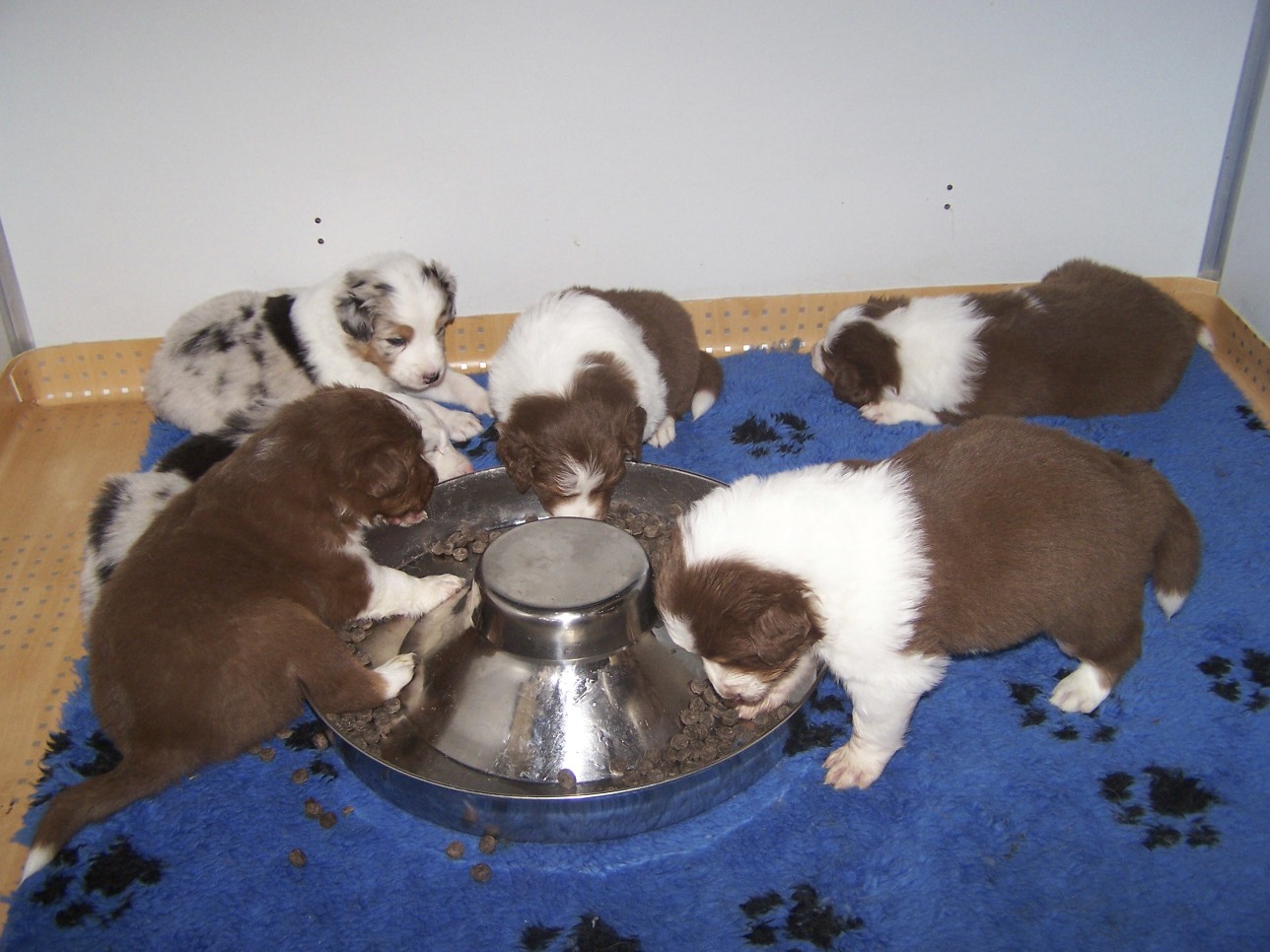The image showcases six young puppies, likely from the same litter, gathered around a large metal feeding dish on the left-hand side. Four of the puppies are predominantly brown with white markings sporadically distributed across their faces and bodies. The remaining two puppies exhibit a mix of colors, including patches of gray, black, white, and hints of brown around their noses and eyes. The puppies appear healthy and well-fed as they eat from the dish. They are all standing or lying on a blue rug adorned with black paw prints, which rests atop an orange grated drainage area. The backdrop is a plain white wall with visible nail holes.